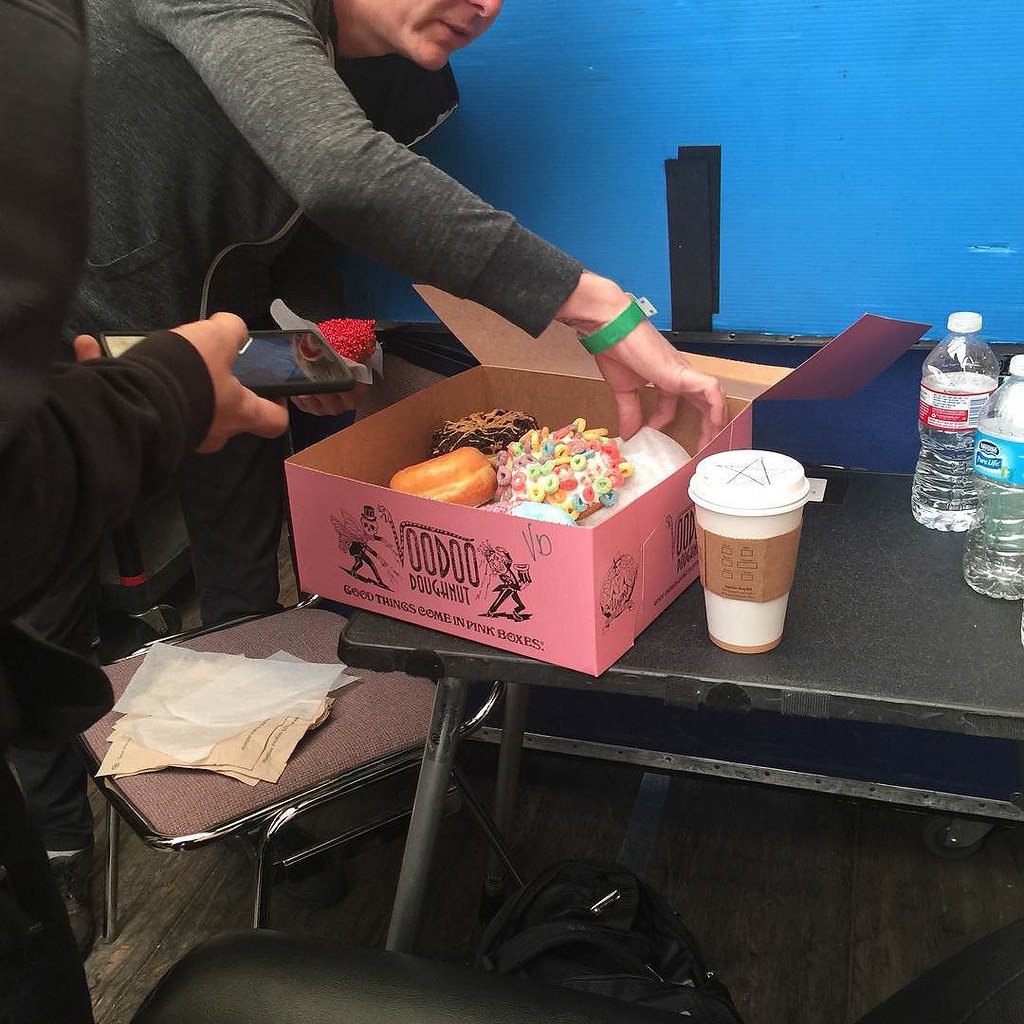In this photograph, we see a lively scene set in a room with a medium bright blue wall. Central to the image is a black folding table with silver-toned legs. On this table sits a distinctive pink box of Voodoo Doughnut, emblazoned with the company's slogan, "Good Things Come in Pink Boxes," and featuring a cartoon mascot of a skeleton with butterfly wings. The box is open, revealing a colorful array of doughnuts, including one with vanilla frosting and Froot Loops, a chocolate-glazed doughnut, and several others partially obscured by wax paper.

Two people are interacting with the doughnuts. One person, wearing a gray long-sleeve top and a green wristband, reaches into the box. The other person, dressed in a black hoodie, stands beside them holding a phone, possibly taking a picture. Also on the table are two water bottles, a white to-go coffee cup with a child-like star drawn on the lid, and a scattering of napkins and bags underneath. The scene is complemented by a chair with a rose-colored tweed seat and a dark gray wood-grain floor, adding to the cozy yet bustling atmosphere.